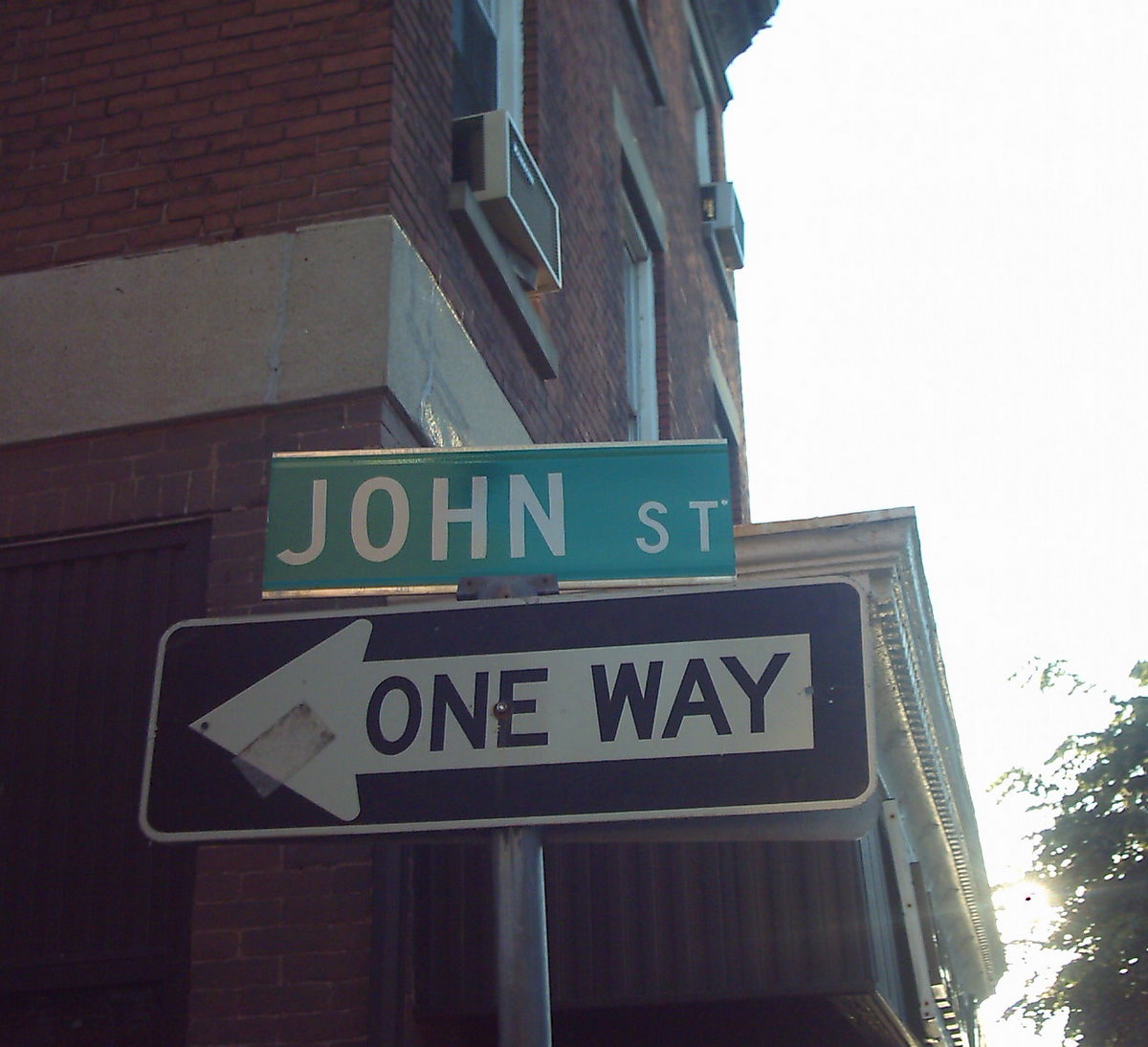The image depicts a street corner with a set of street signs. The top sign is a standard green rectangular street sign with the name "John Street" displayed in large white letters. Directly beneath it is a one-way directional sign, which is also rectangular. This sign features a black inlay with a white border and a white arrow indicating the direction, accompanied by the words "One Way" in black text.

Behind the signs, there is a brick building that appears to be residential or possibly an office, as evidenced by the multiple air conditioning units visible in the windows. In the lower right corner of the image, the edge of a tree is partially visible. The lighting suggests that the photo was taken during twilight, either dawn or dusk, when the light conditions are dim and create a grayish atmosphere, making it neither too bright nor too dark.